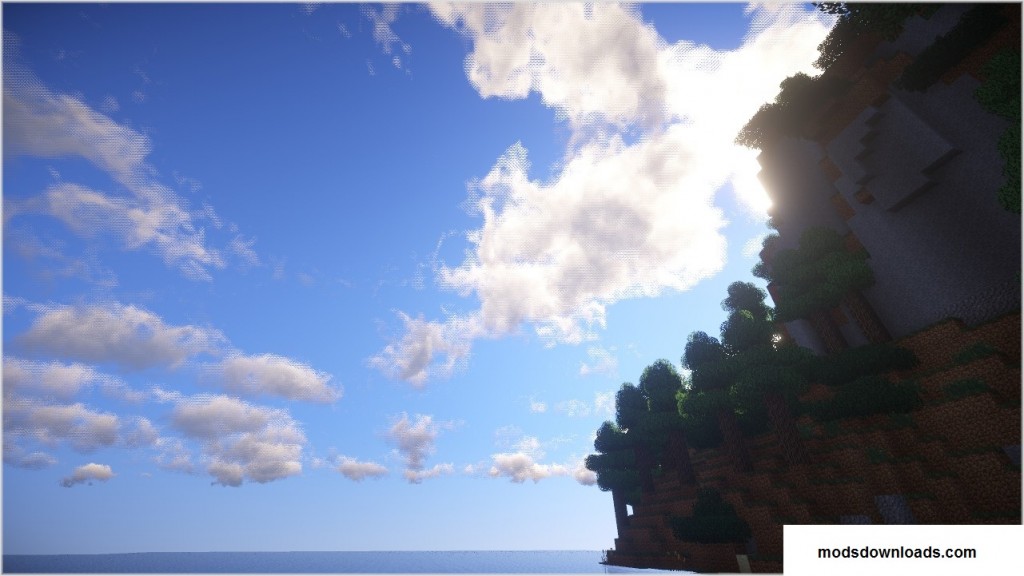This digital image, likely from a video game such as Minecraft, features a vast and captivating scene. Dominated by a beautiful blue sky scattered with thick white clouds, the horizon sits prominently at the bottom of the frame. On the top right, the sky is especially bright, with the sun illuminating the scene through layers of clouds. The right side of the image showcases a gray and brown colored stone cliff or structure, with an adjacent hillside covered in green trees and brown hedges, resembling a maze. The land meets the waters of an ocean or large body of water, which spans from the bottom right to the bottom left of the image. The water's edge is marked by the text "mods downloads com" in a white bar with black text on the bottom right corner, adding a digital touch to the scene. This serene and vividly detailed landscape captures the essence of a crafted virtual world.